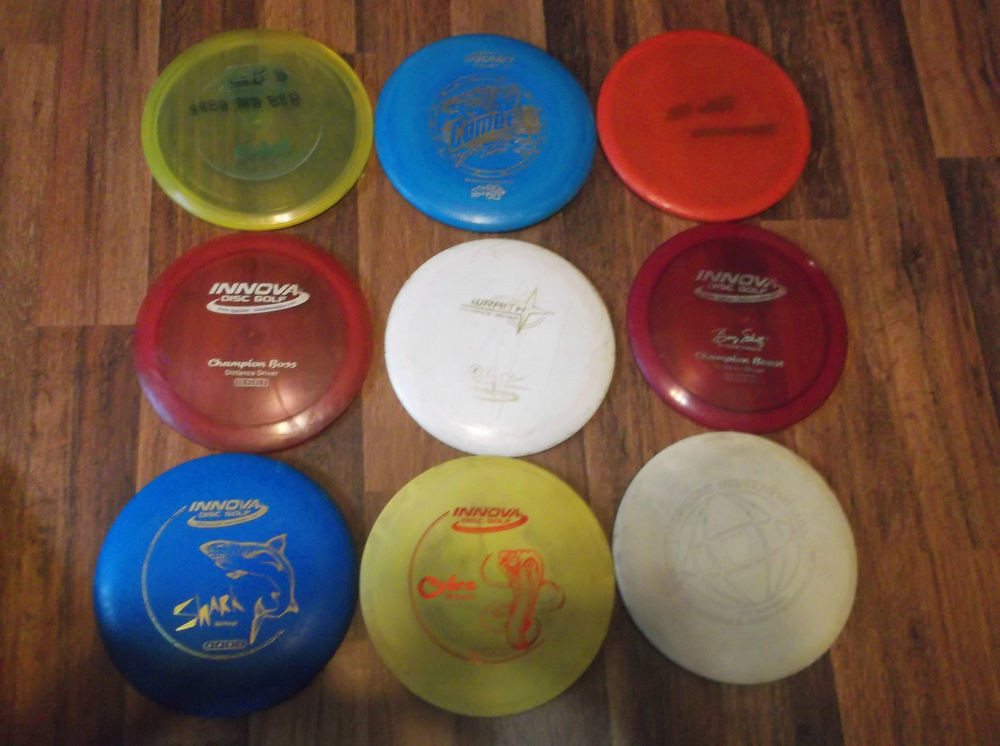This image features nine well-used disc golf frisbees arranged in a grid pattern on a medium to dark brown hardwood floor. The frisbees are displayed in three rows of three, viewed from above. Starting from the top left, the first row includes a translucent yellow frisbee with unreadable faded black writing, a solid blue frisbee with gold writing, and an orange frisbee. The second row has a red translucent disc labeled "Innova Disc Golf Champion Boss," a white frisbee with faded gold writing, and another translucent red Innova disc. In the bottom row, there's a blue Innova frisbee with gold lettering and a shark image, a yellow Innova disc featuring a cobra imprint in red, and an off-white frisbee with indistinct markings due to wear. The prominent brand on most of these frisbees is Innova, known for their disc golf discs.